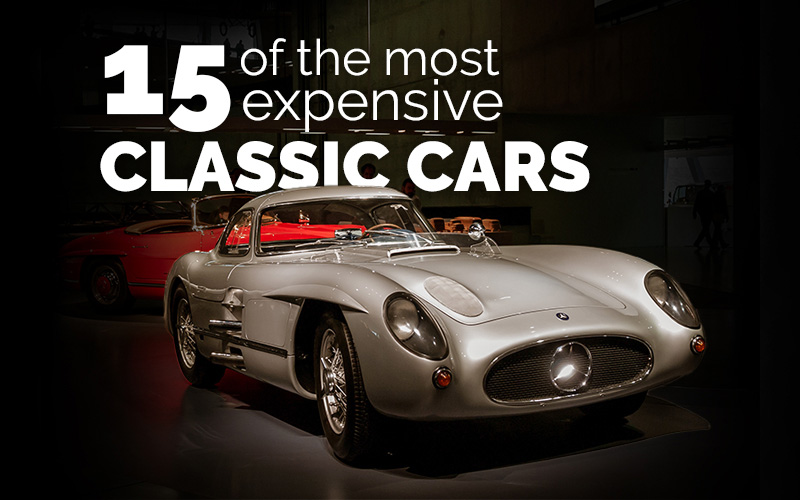This image captures a silver classic sport car, likely a Mercedes, positioned at an angle in the foreground. The car features two narrow oval headlights, red taillights, and chrome wheels, and is set against a dark gray background that includes its shadow on the floor. Above the vehicle, white text reads "15 of the most expensive classic cars." Behind the silver car, a red convertible is partially visible, revealing its roofless design, hood, and some seating. The photograph, which emphasizes the front and side profile of the Mercedes, is rich in colors including black, white, dark gray, light gray, silver, and red, although the exact setting remains indeterminate.